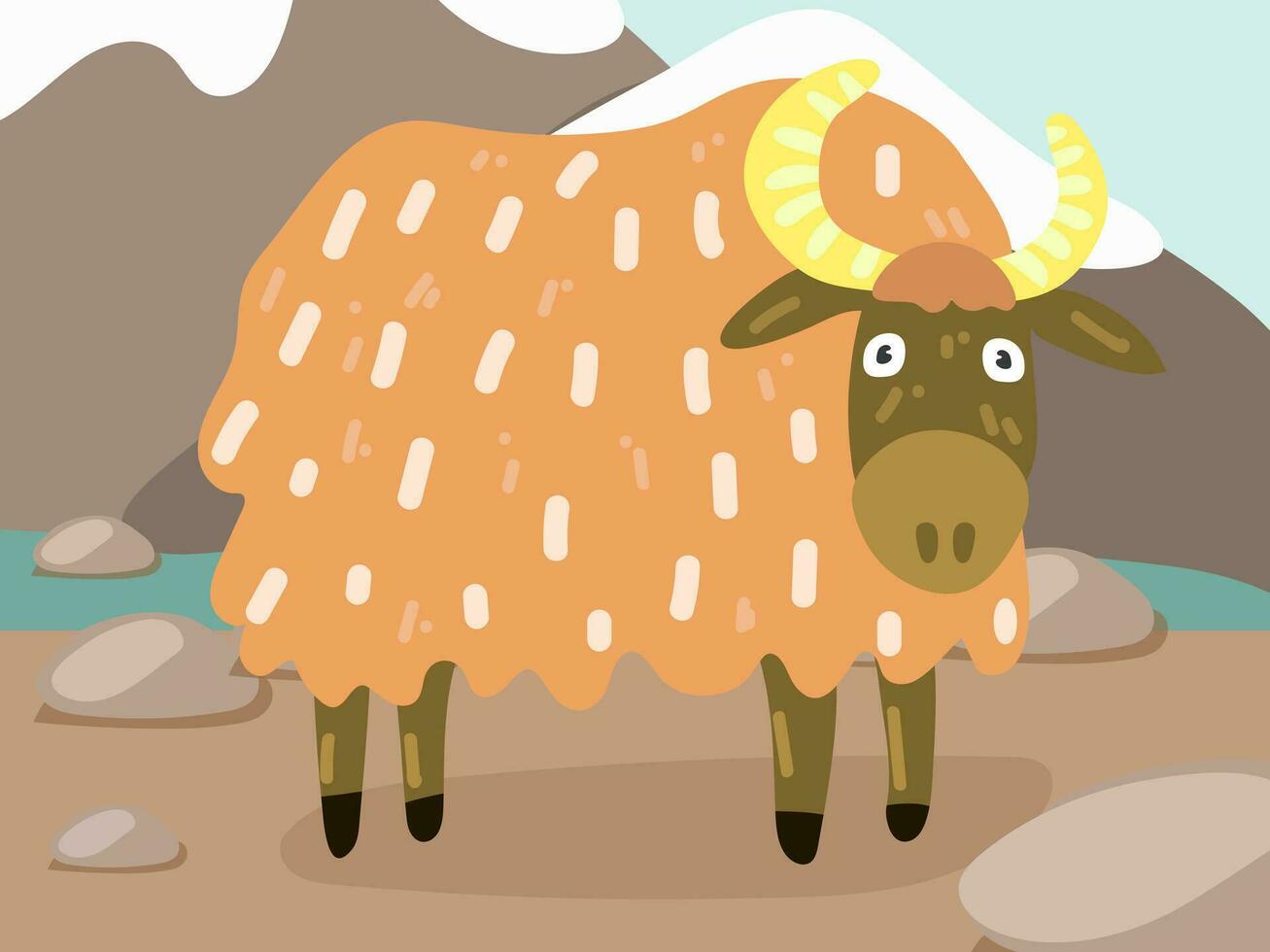This image features a modern-day, cartoonish drawing of a bull characterized by its adorable and stylized appearance. The bull has a light orange coat adorned with oval patterns, and boasts a brown face, ears, and legs. This charming creature also has a tan patch on the top of its head, large black eyes set against a backdrop of white, and a big, cute nose. The bull's horns are yellow with lighter yellow lines, adding to its detailed and whimsical appeal. Standing on a rocky, brown ground, the bull is positioned in front of two contemporary, cartoon-like mountains with white snowcaps. There is a small pool of turquoise water just below the mountain backdrop, enhancing the picturesque and modern design of the scene.